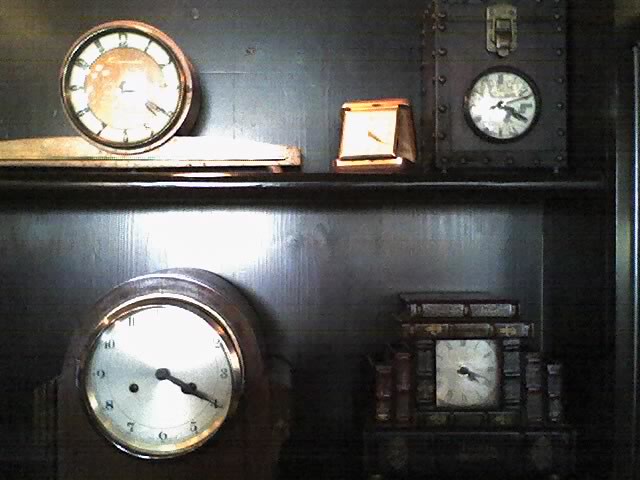In this image, there are five clocks displayed on a shelf with three on the top row and two on the bottom. The photo quality is somewhat grainy, and the lighting tends to wash out the details. The top left clock has a circular face with a copper frame. The middle clock on the top row resembles a large square-faced watch. To its right, there is another circular clock, encased in a locked container. On the bottom row, the left clock is circular, while the one on the right appears to be a square clock, partially obscured by several books.